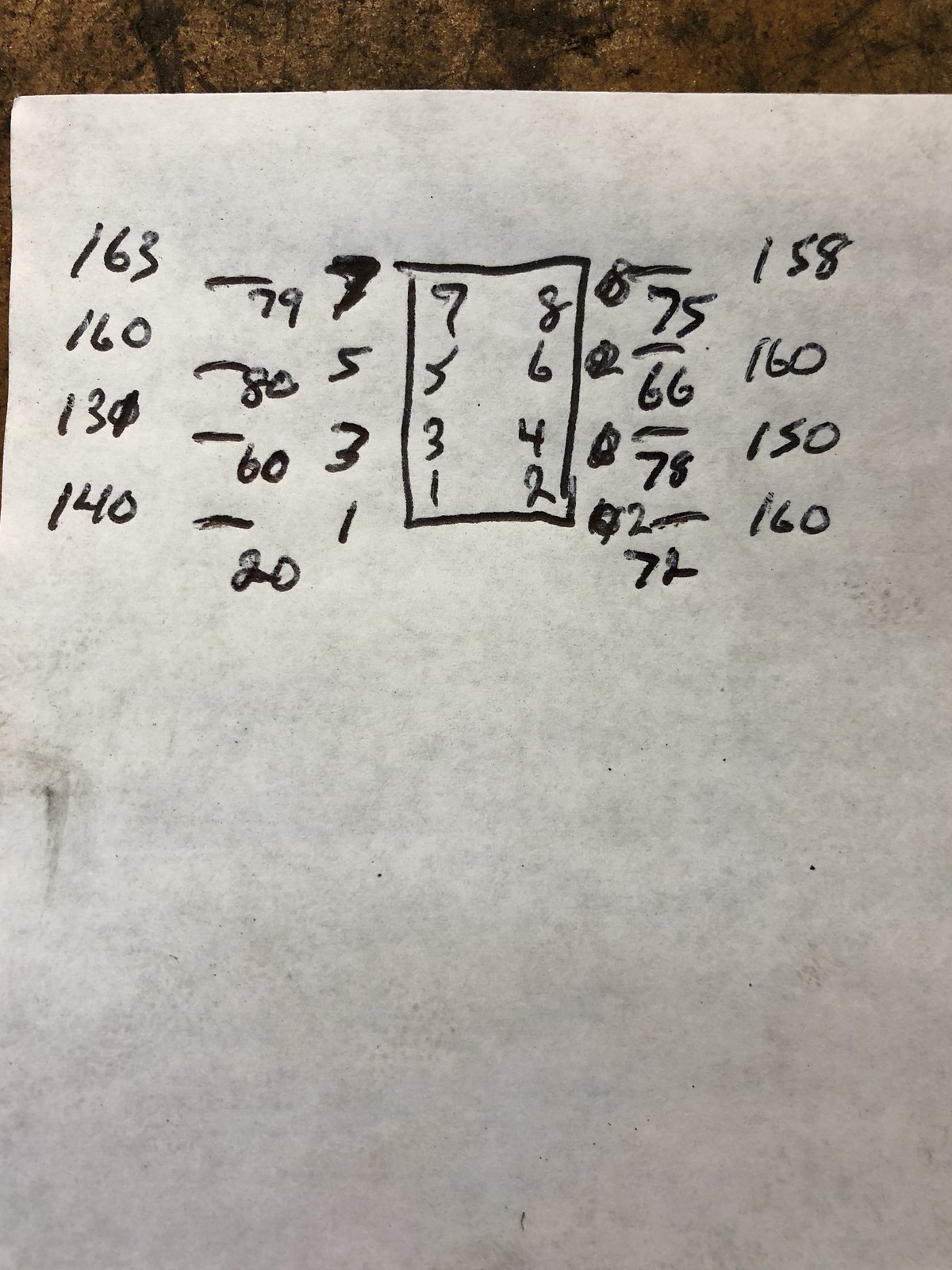The photograph displays a sheet of paper covered in scrawly black ink handwriting, likely made using a thick ballpoint pen. The writing consists of an assortment of random numbers organized into various columns and one central box. On the leftmost column, running from top to bottom, are the numbers 163, 160, 131, and 140, each separated and lined off. Moving right, the next column contains the numbers 79, 80, 60, and 20. 

Further right, central to the sheet, is a tightly framed box with two vertically aligned columns inside displaying the numbers 7531 and 8642. Adjacent to this box and towards the right, another column lists 75, 66, 77, and 72. On the far right, there's yet another column featuring the numbers 158, 160, 150, and 160. Notably, an additional column has been scribbled out entirely, making the numbers illegible.

The handwritten numbers and columns are irregular and appear hasty, with evidence of the pen skipping and creating broken lines on the paper. The overall impression is of a very messy and untidy document, possibly serving as a record for weight loss or a similar tracking method. The writing style hints at a young individual, perhaps a teenager, due to its disorganized and somewhat erratic nature.